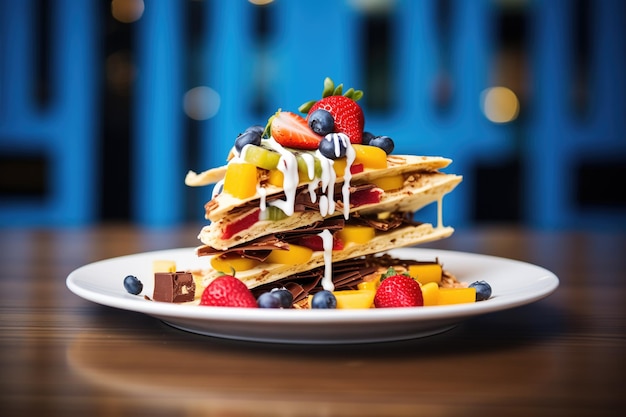An artfully posed photograph showcases a multi-layered tart presented on a white plate, which rests on a brown table. The background is a blurred electric blue, devoid of distinguishing features. The tart itself is composed of thin baked tortillas or bread slices, each layered with a medley of fruits and chocolate. The fruit toppings include a vibrant mix of sliced and whole strawberries, blueberries, as well as pieces of peach or mango, and some light green kiwi or bits of pineapple. Additionally, finely shaved chocolate is interspersed among the layers, and a white cream-like frosting drizzles elegantly over the tart, cascading towards the plate. To the left on the plate, there is a significant chunk of chocolate. Scattered around the base of the tart are miscellaneous whole blueberries and strawberries, adding to the dessert's detailed and delectable presentation.